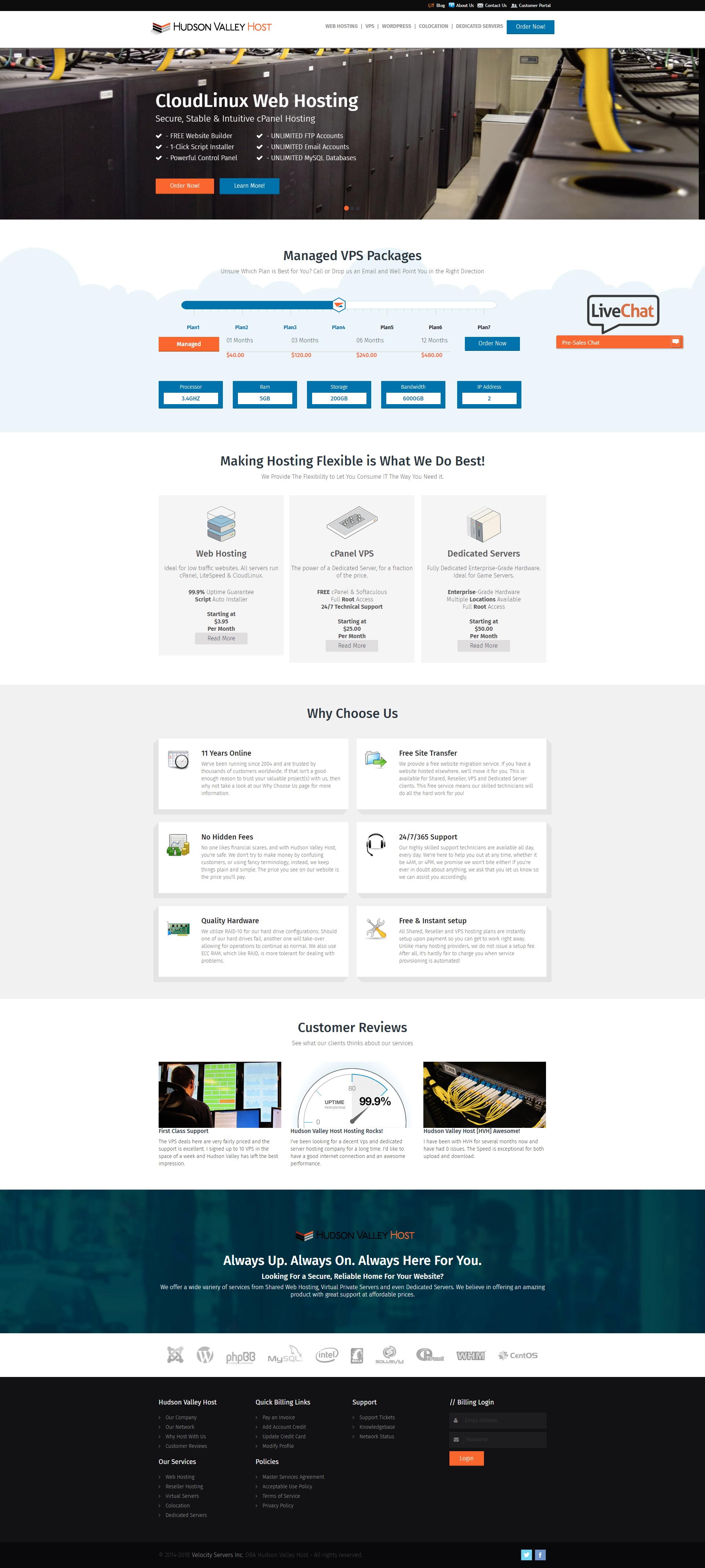The image in question is a vertically-oriented screenshot of a website, approximately two and a half to three times taller than it is wide. The layout captures the entirety of the webpage, but the compression makes it challenging to discern the finer details, especially the smaller fonts.

### Detailed Descriptive Caption:
The top section of the image features the website's logo, occupying about 20% of the width. The logo depicts a pair of stylized wings, reminiscent of military insignia—black on the left and gold on the right. To the right of the logo, the text "Hudson Valley Host" is barely legible. Adjacent to the logo, a horizontal menu bar stretches across the top-right corner, comprising approximately five menu options. A distinctive blue button is positioned at the very top of this menu.

Immediately below the header, a banner spans roughly the next 15% of the image’s height. The banner’s background appears to be an aerial view of computer hardware, suggesting a server room environment. Superimposed on this background in white text is the phrase "Cloud Linux Web Hosting." 

Below this headline, two columns of text are visible, but their minute size renders the details unreadable. Each column contains three bullet points, totaling six points of information. Anchoring this banner are two prominent buttons: one orange button on the left side and a blue button on the right side.

### Summary:
The website screenshot’s dense vertical orientation compresses the layout, incorporating a logo, navigation menu, and a banner with a background image of server hardware. The banner promotes "Cloud Linux Web Hosting" with accompanying bullet points and action buttons, presented in a visually structured format.